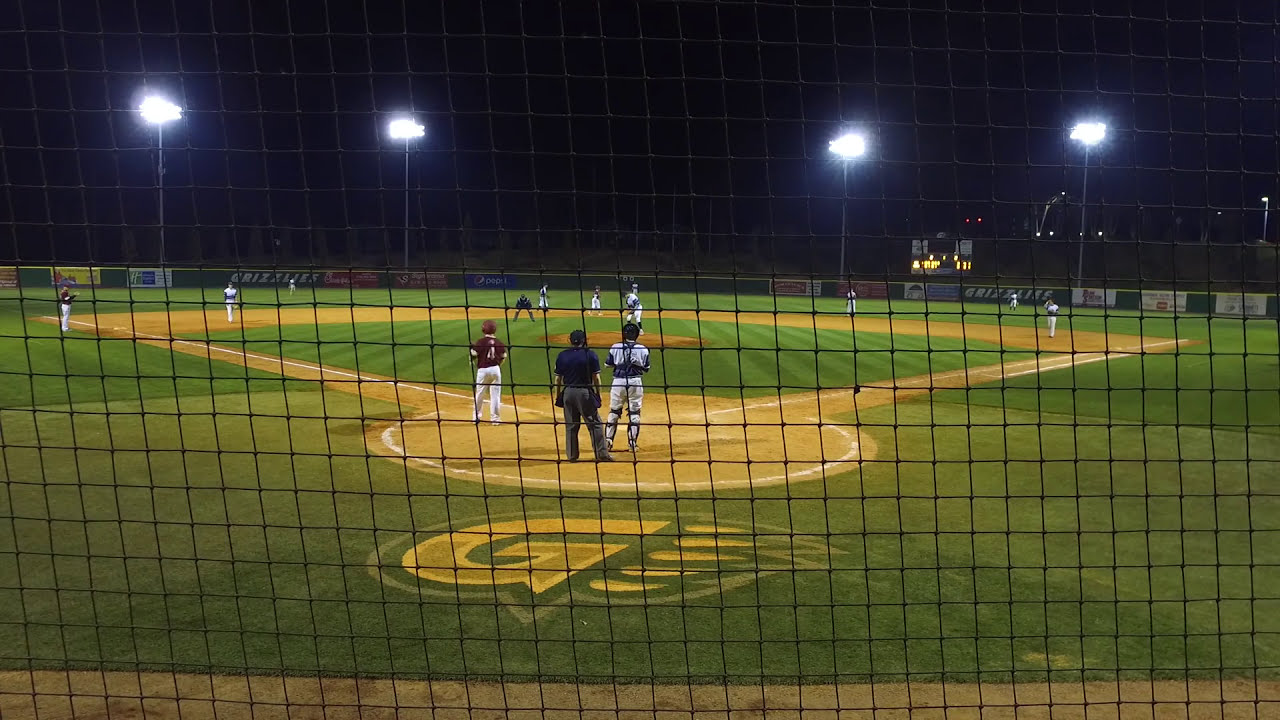This is a detailed nighttime photograph of a baseball game, likely a high school, college, or minor league event. The image is captured from behind the backstop netting, which appears as a grid of squares in the foreground. The scene centers on a batter's box to the left, where a player from the batting team, dressed in maroon shirts, white pants, and maroon helmets, is awaiting the pitch. The fielding team, clad entirely in white, is positioned defensively on the green field, with a runner standing on second base. 

The catcher is up from his crouch, while the umpire is positioned behind him at home plate. In the distance, the pitcher stands motionless on the mound. The infield's brown dirt contrasts with the verdant grass, which features letters and a logo—a capital 'G' with flame or claw-like designs pointing to the right—etched into it. 

Bordering the field are several low walls adorned with advertisements, with a scoreboard illuminated against the dark sky. The night scene is brightly lit by four towering floodlights, two on each side of the field, casting a broad glow over the action below. The atmosphere is calm and paused, capturing a moment of stillness in the game.